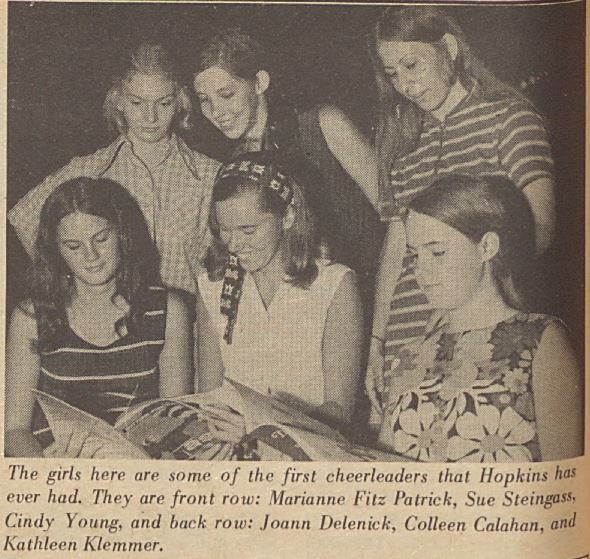This old, square newspaper clipping features a yellowed black-and-white photograph of six young women, identified as some of the first cheerleaders at Hopkins. The image is discolored with age, giving the paper an off-white, orangish hue. In the front row, seated, are Marion Fitzpatrick, Sue Steingrass, and Cindy Young; they appear to be focused on magazines or pamphlets in their hands. Standing behind them, looking over their shoulders, are Joanne Delanick, Colleen Callahan, and Kathleen Clemmer. All the girls have long hair, and while most are smiling, they are all engaged with the reading material. The photograph reflects the fashion style of the 1960s or 1970s. Below the photo, the newspaper caption lists their names by rows, noting the historical significance of this cheerleading team at Hopkins.